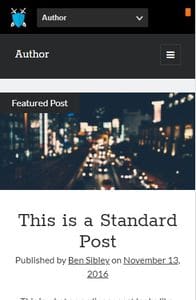This small, pixelated screenshot appears to be from a mobile phone. At the top is a black bar with a blue shield icon on the upper left, featuring two gray swords crossed behind it. To the right of the shield is a gray rectangle with the word "Author" in white font, accompanied by a drop-down arrow. The upper right corner displays a small green square.

Below the black bar, there is another gray rectangle with "Author" on the left in white font, and a small outlined square with three horizontal lines stacked vertically to the right. This is followed by a white bar, leading into a low-quality photo of a bustling city street at night, filled with lights in the darkness. In the upper left corner of the photo, there is a gray box with the text "Featured Post." 

At the bottom of the image, on a white background, it reads "This is a standard post" in black font.